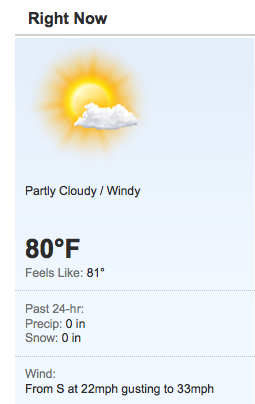**Detailed Weather Page Snapshot:**

This weather webpage falls under the "websites" category and features a simple, light gray background. Dominating the upper-left corner of this background is a vivid and bright digital rendering of a sun with numerous rays emanating outward. The sun's core is intensely bright, and the rays gradually fade as they extend outward. A fluffy white cloud sits in front of the sun, partially obscuring it. 

Beneath this graphical representation, bold black letters read "Partly Cloudy / Windy" along with the current temperature displayed prominently as "80°F" in bold, large font, accompanied by a smaller note indicating it "Feels like 81°F." Additional weather statistics are listed below this main information:

- Precipitation over the past 24 hours: 0 inches
- Snowfall over the past 24 hours: 0 inches (humorously noting that it's unlikely given the 80°F temperature)
- Wind: Coming from the South at 22 miles per hour, gusting up to 33 miles per hour

This concise block of weather information provides a quick glance at the day's weather conditions without offering details on its source, whether it’s from AccuWeather, The Weather Channel, or a local news station.